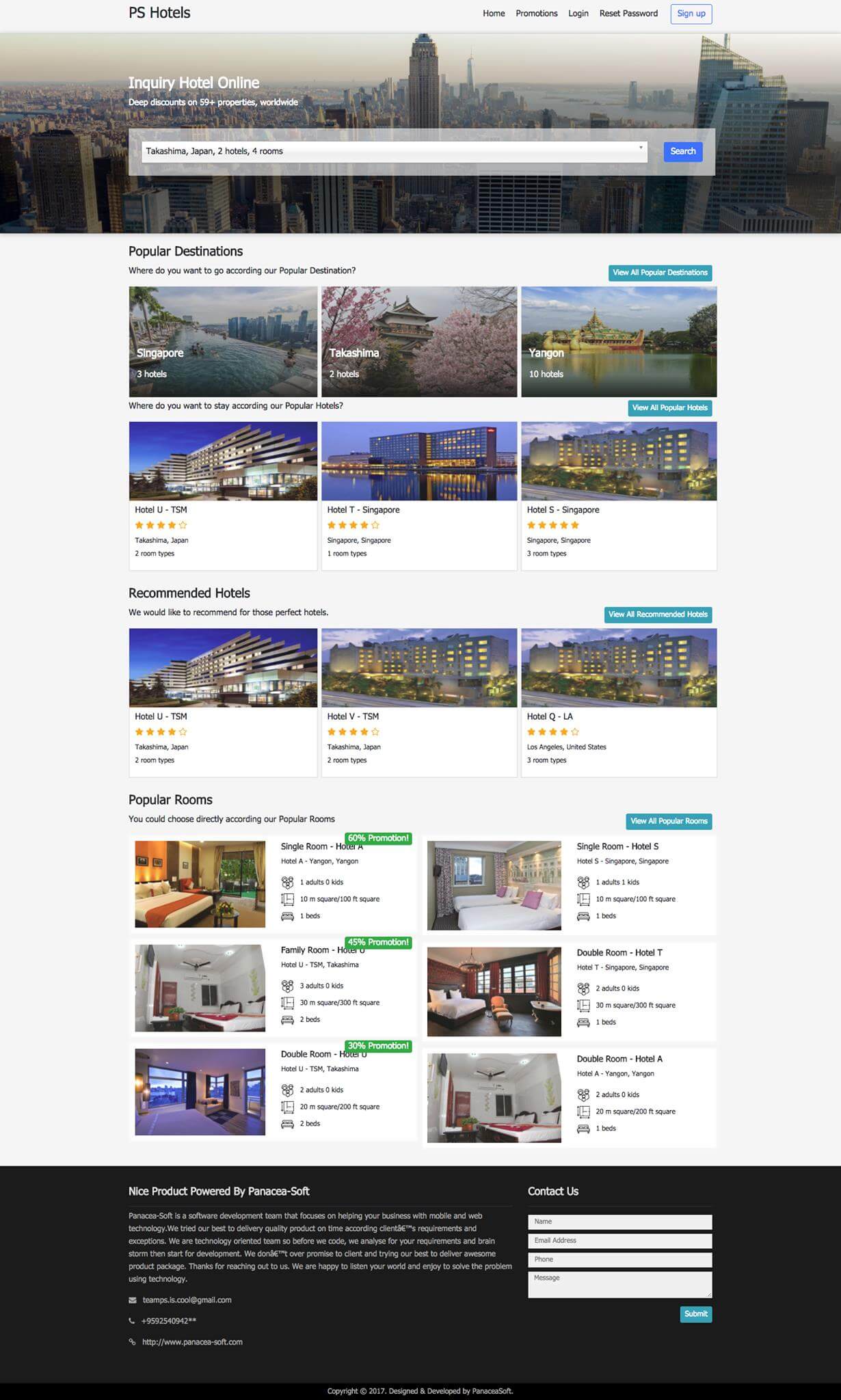Here is a cleaned-up and detailed caption for the described image:

---

The screenshot from the website showcases a user-friendly interface with a light-gray banner at the top. The banner prominently features the text "PS Hotels" with "NPS" in capital letters, followed by the word "Hotels" also capitalized, all in black typeface. On the right-hand side of the banner, navigation options titled "Home," "Promotions," "Login," and "Reset Password" are visible, along with a clickable "Sign Up" option.

Beneath the banner, the screenshot displays a serene cityscape, complete with buildings, sky, and a body of water. A search bar is positioned below the imagery, featuring the text: "Inquiry Hotel Online - Deep Discounts on 59+ Properties Worldwide." Within the search bar, the query reads: "Takashima, Japan - 2 Hotels, 4 Rooms," accompanied by a blue search button on the right-hand side.

As the page continues, it introduces a section titled "Popular Destinations," set against a white background, and includes six images with destinations such as Singapore, Takashima, and Yangon, each linked to their respective hotels. The next section is labeled "Recommended Hotels," where the website suggests three hotels deemed perfect for users, inviting them to explore these recommended options.

Further down, the website highlights "Popular Rooms," providing three choices on the left and three on the right side of the screen. 

At the bottom of the page, a footer reads "Nice Product Powered by Panacea/Soft," followed by detailed contact information including email, phone number, and the website link.

---